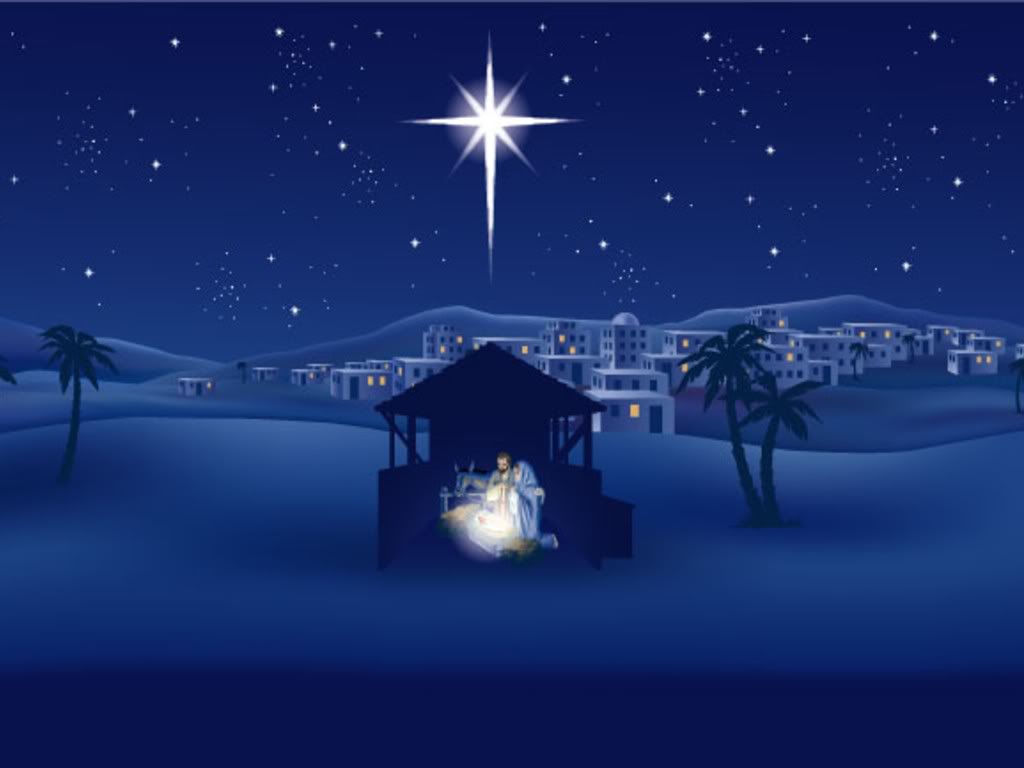The illustration portrays a serene night scene of Bethlehem, a historical Middle Eastern village. Central to the composition is a humble manger, symbolically depicting the birthplace of Jesus Christ surrounded by the modest architecture of ancient Bethlehem. Above the scene, nine stars twinkle against the darkened sky, with one particularly luminous star dominating the celestial expanse, likely representing the Star of Bethlehem. The color palette is limited yet evocative, featuring deep blacks, tranquil blues, and radiant whites, capturing the mystical and sacred nature of this pivotal moment in Christian lore.